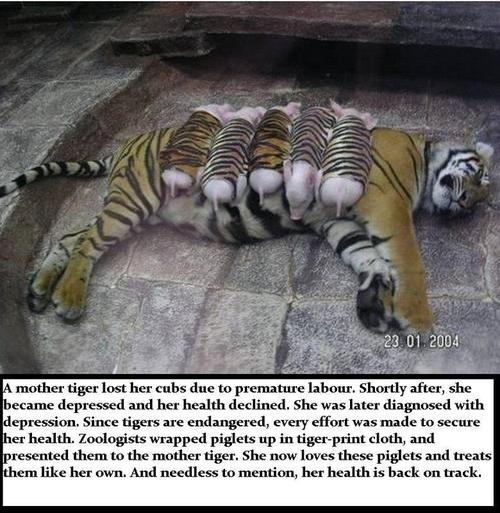This square image, dated January 23, 2004, captures a poignant moment of a female tiger lying on her left side on a stone floor, possibly in a zoo enclosure. She sports the distinct pattern of a tiger: a white stomach with black stripes, and the rest of her body covered in brown fur with black stripes. Her visible right side of the face highlights white with stripes and some brown on top. Draped across her body are five piglets, swathed in cloth designed to mimic tiger fur, making them appear as if they seamlessly belong to her. The text at the bottom informs us that this mother tiger fell into depression and her health declined after losing her cubs due to premature labor. To uplift her spirits, zoologists ingeniously wrapped piglets in tiger-patterned cloth and introduced them to the mourning tiger. Accepted as her own, the tiger's health dramatically improved as she nurtured these unlikely surrogates, treating them with the love and care she had yearned to give her lost cubs. The heartwarming story is underscored by the background, which suggests a controlled environment such as a zoo, reiterating the lengths taken to ensure the well-being of this endangered creature.